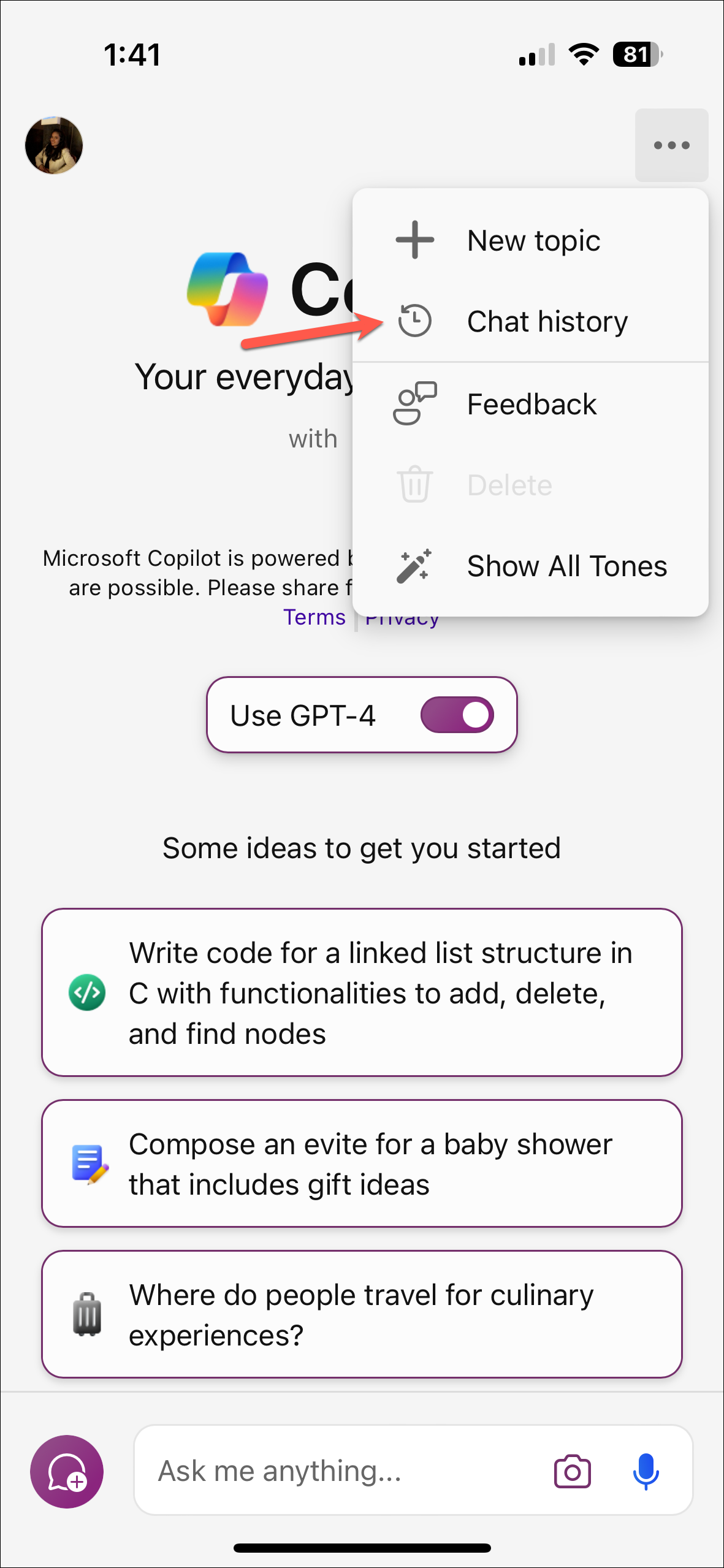Screenshot of a website interface featuring a sleek gray background. At the top, in bold black text, the time is displayed as "1:41". To the right of the time are icons indicating a strong signal strength, Wi-Fi connectivity, and an 81% battery level.

On the left side of the screen, there's a circular profile picture of the user. Adjacent to this is a colorful graphic resembling a rainbow-shaped arc. Below the arc is the text "Your everyday," which appears to be a truncated message or heading.

A popup window overlays the main screen, featuring a plus sign icon next to the text "New Topic" in bold. The popup also includes a clock icon labeled "Chat History" with a prominent red arrow pointing to it. Further down, there are options for "Feedback" and a grayed-out, inaccessible "Delete" option.

The popup continues with a "Show All Tones" button, marked with a magic wand icon. "Use GPT-4" is switched on, and beneath it, a list of suggested ideas to get started is displayed:
1. Write code for a linked list structure and see what functionalities to add, delete, and find nodes.
2. Compose an e-vite for a baby shower that includes gift ideas.
3. Explore popular culinary travel destinations.

At the bottom of the popup, there is a small circle with a speech bubble containing a plus sign labeled "Ask me anything," accompanied by camera and microphone icons.